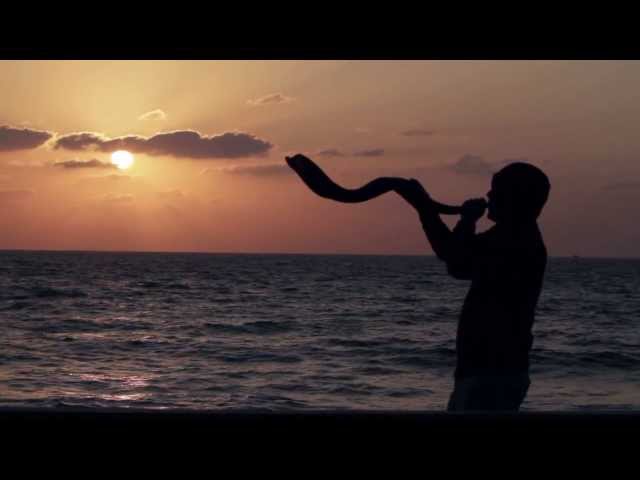This landscape-oriented photograph captures a stunning sunset on the beach. The setting sun sits just off to the left, casting a radiant golden hue with hints of pink and orange across the sky. A few streaky, dark gray clouds hover above, adding drama to the vibrant scene. In the background, the slightly wavy ocean stretches out, reflecting the descending sunlight. Towards the bottom of the image, the ocean meets a black border, enhancing the silhouette of a man positioned in the right corner. Dressed in unidentifiable clothing, he holds an intricately wavy, possibly wooden horn to his mouth, appearing to play or prepare to blow into it. The photograph, slightly blurry but still captivating, beautifully combines elements of light, color, and silhouette to create a memorable and atmospheric moment at the beach.